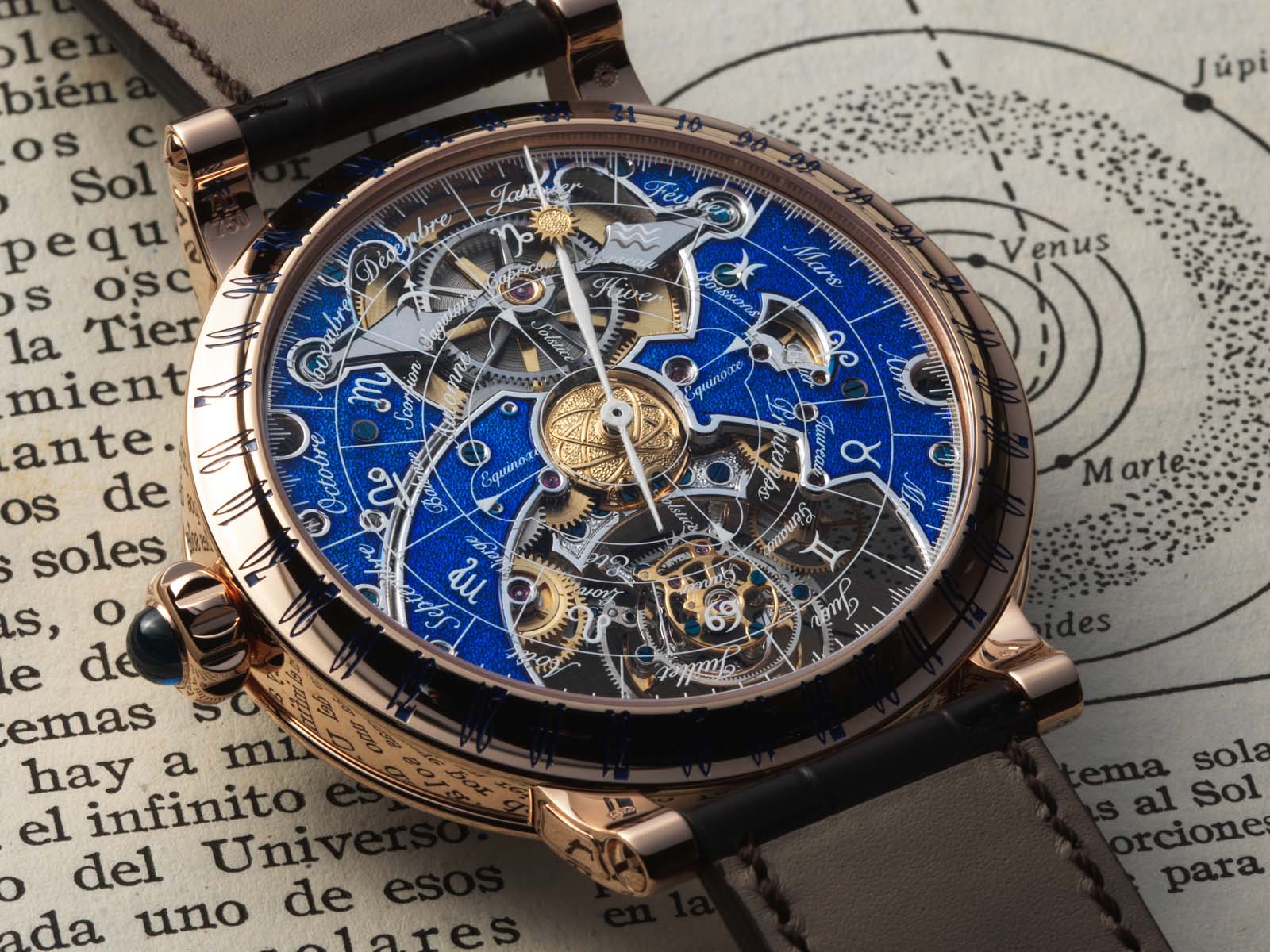The photograph showcases a highly intricate and luxurious wristwatch set against a backdrop with astrological diagrams. The watch itself features a rose gold casing with a clear glass face and back, revealing its complex inner workings, including visible gears. One of the hands of the watch is particularly distinctive, adorned with a small golden sun at its tip. This hand appears to function as a guide for constellations, moving across an elaborately designed dial that includes both astronomical symbols and months of the year. The watch face, with a rich blue background, is surrounded by numbers and gauges, enhancing its ornate appearance. Encircling the center, a dial extends from the outer edge to a quarter of the circle, possibly indicating specific astrological or chronological data. The timepiece is secured by a brown leather wristband and is positioned atop papers or a book that prominently feature astronomical maps and charts. This intricate wristwatch blends elements of timekeeping, astrology, and astronomy, making it a unique and sophisticated piece perfect for enthusiasts of celestial navigation and horology.